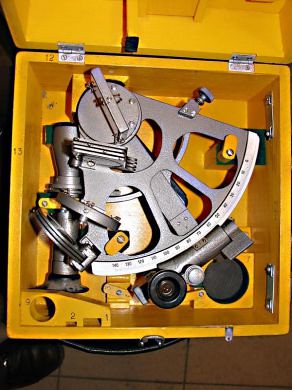The image depicts a precision instrument encased in a custom-fitted yellow storage case with silver hinges. The device inside, which appears to be either a gyroscope or a theodolite, is a complex metal apparatus likely used by surveyors or similar professionals. The instrument is a dark silver metallic color with various black lenses and numerous adjustment mechanisms, including a carved dial whose intricate details are not fully visible. The interior of the case is meticulously cut to accommodate each component of the instrument perfectly, ensuring secure storage. The yellow case is open, revealing the snug fit of the device, and below it, a man’s foot is visible against light-colored floor tiles, adding a subtle human element to the scene.